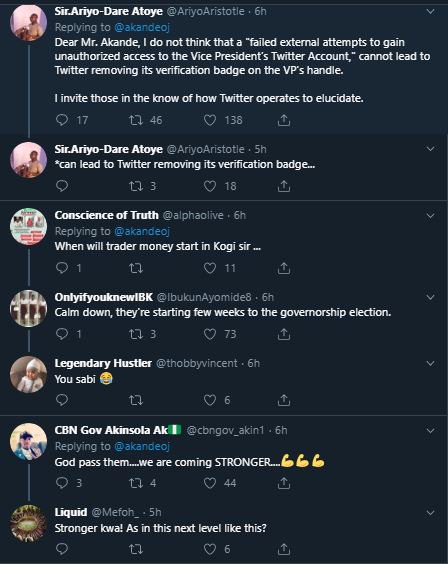This is a screenshot of a tweet thread, captured from an iPod, evident by its wide, square aspect ratio rather than a thinner, rectangular one. The screenshot showcases seven comments replying to an original post, although the post itself is not visible. 

Each comment follows a structured layout:

- On the far left side of the screen, user profile pictures are displayed.
- To the right of each profile picture, the user’s name appears. 
- Following the username, in a light gray color, is the user's handle.
- Adjacent to the handle is the time indicating how long ago the tweet or reply was made.

Beneath each user’s name, it states "replying to," followed by the handle of the user they are replying to, highlighted in blue.

The background of the screenshot is black, indicating the device is in night mode. On the far right side of each comment, there are arrow buttons pointing downwards, enabling users to collapse and minimize individual comments.

At the bottom of each comment, there are four interactive icons:

- A chat bubble icon for replying.
- An arrow icon resembling a retweet symbol.
- A heart icon for liking the comment.
- A share icon for sharing the comment.

This detailed layout provides a comprehensive view of the conversation, ensuring ease of navigation and interaction within the Twitter thread.